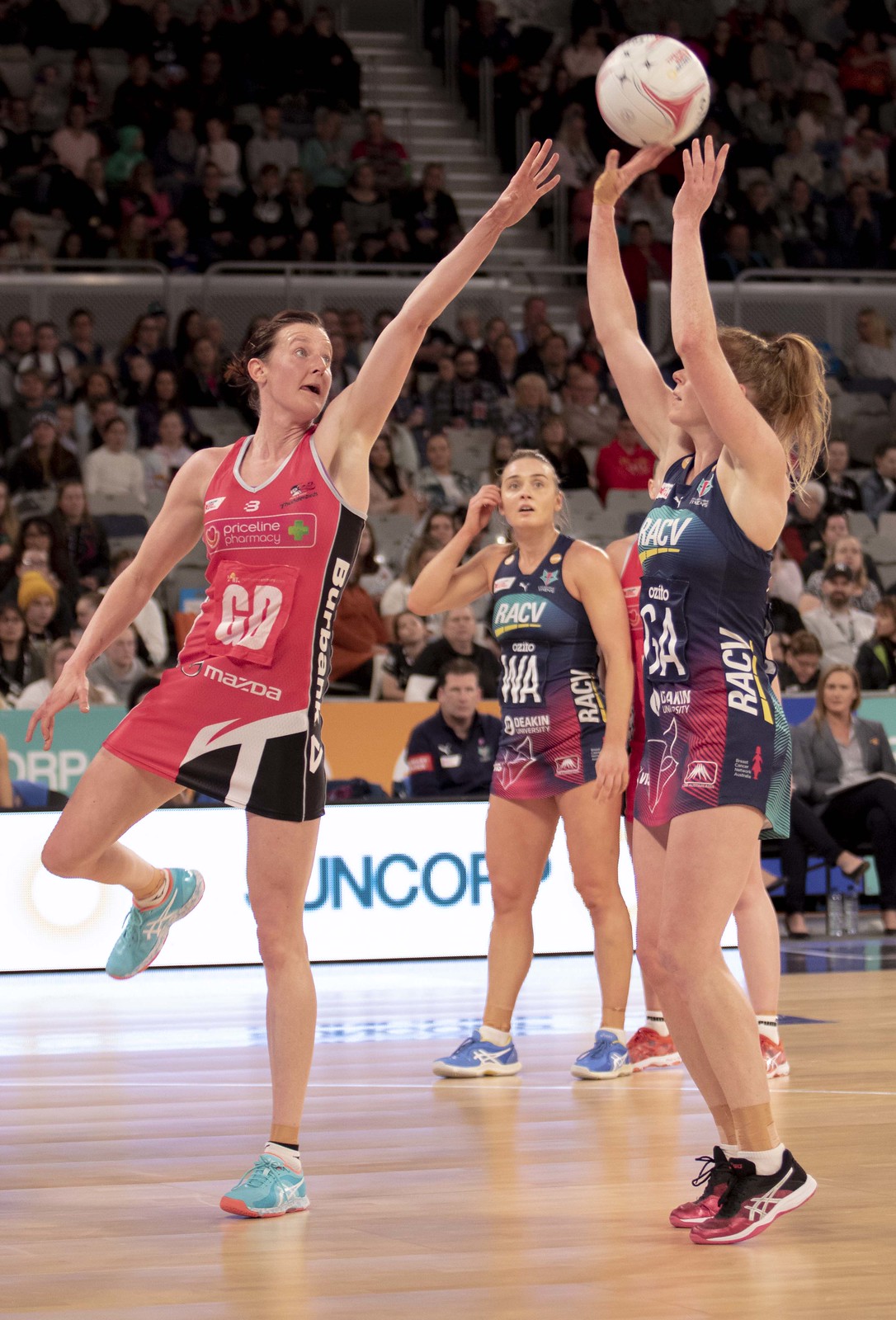In this dynamic and action-packed photo taken directly on the court during a women's volleyball game, four players are in the midst of a play. Two players, wearing dark blue spandex tank tops and skirts with red and white lettering, are attempting to control the ball. One of them is on her tippy toes with her arms fully extended above her head, fingertips just touching the ball. The other player in blue has one foot firmly planted on the ground and is reaching out towards the ball as well. The other two players, dressed in red and black outfits similarly styled, are intensely focused, with one of them also reaching out towards the ball, trying to intercept it. The court's polished light brown wooden floor is clearly visible beneath the players. In the background, there are two tiers of raised bleachers filled with hundreds of spectators, eagerly watching the game. Additionally, a long table draped with a white banner that reads 'UNICORP' in blue lettering can be seen along the sideline, partially obscured by the movement of the players.